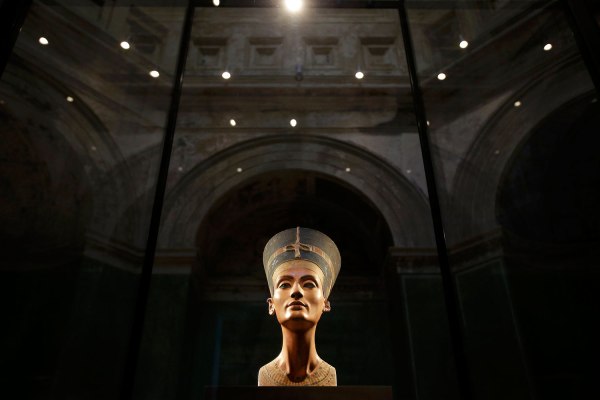The image depicts the famous head sculpture of Nefertiti, housed in a glass case within a museum. The surroundings, captured in dark and muted tones of gray, black, and muddy brown, suggest a grand, historical building, possibly an ancient castle or a renowned museum like the Louvre. The background showcases large archways, adding to the majestic atmosphere. The Nefertiti sculpture, centered prominently towards the lower middle of the frame, is bathed in focused light, emphasizing its exquisite details and stoic expression. The headdress, reminiscent of an upside-down lampshade, is distinctly highlighted. The setting appears empty, creating an intimate moment with the famed artifact, as if being observed alone.